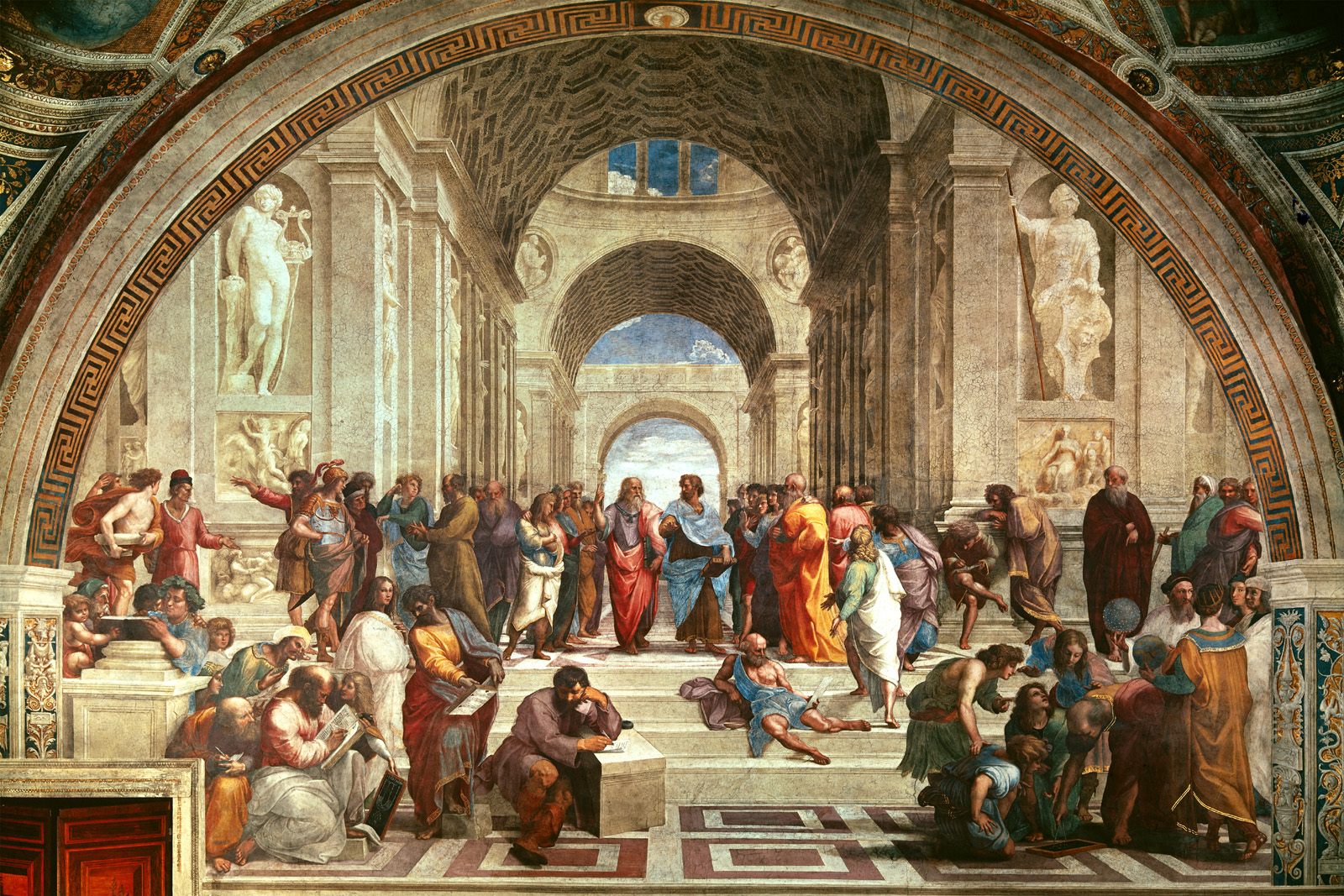This detailed painting, known as "The School of Athens," is a Renaissance fresco depicting an assembly of ancient philosophers, composed around 1509-1511 by Raphael. Set under a grand arched marble structure, it captures dozens of figures, predominantly men in colorful robes of blue, red, white, brown, and orange, spread across a series of steps. In the foreground, figures sit, stand, and recline on the steps, engaging in animated discussions. Notably, at the center of the composition, Plato and Aristotle stand in an iconic pose, likely pointing towards their philosophical debates. Surrounding them, groups of people are immersed in activities such as writing, thinking, and conversing. The marble flooring features a white and maroon blocky pattern, leading up to a series of receding arches opening onto a bright, white sky. The painting’s background also houses intricate ornamentation and statues integrated into the architecture, elevating the grandeur of this classic portrayal of intellectual exchange.